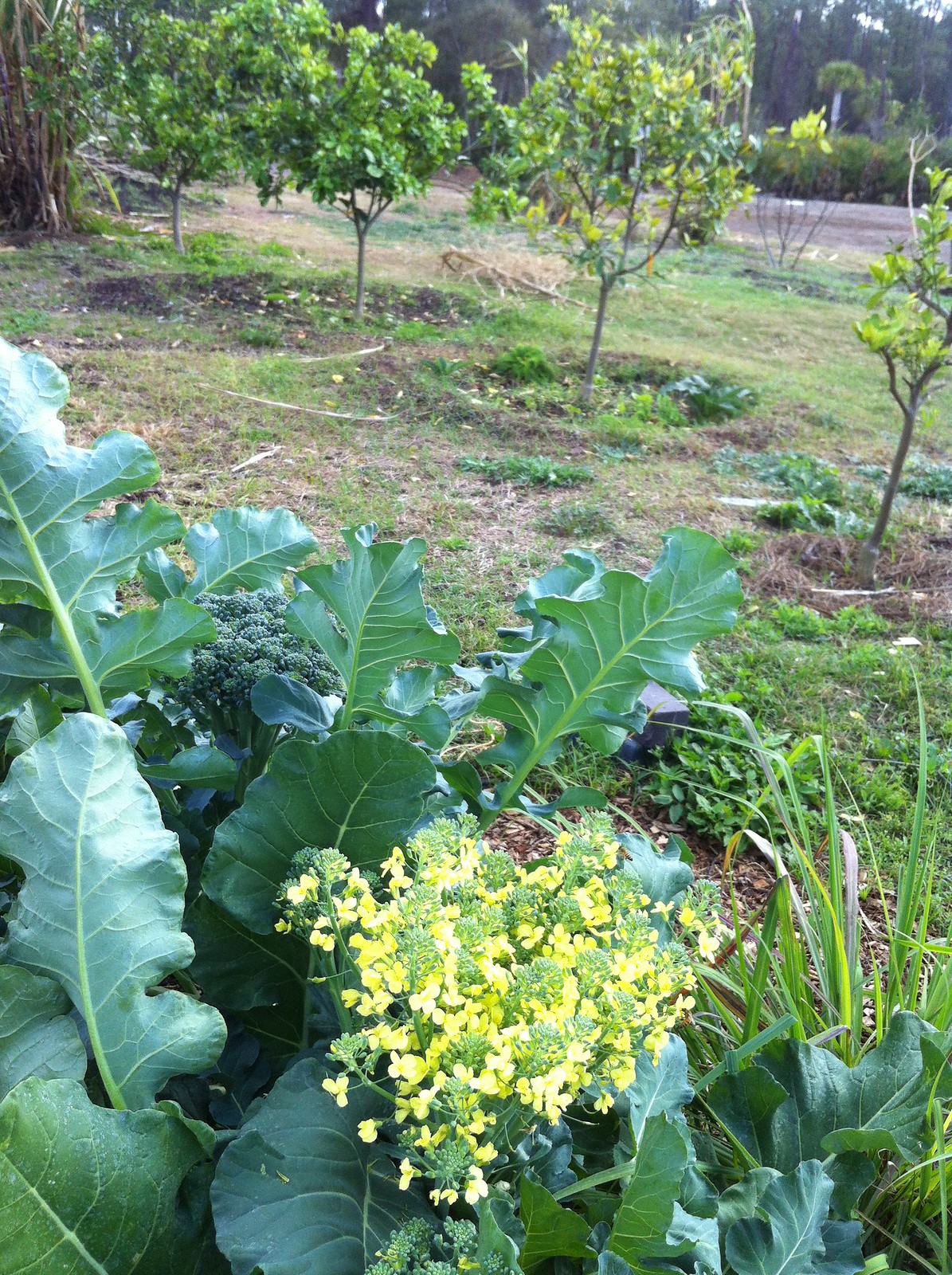A garden scene featuring lush, large green leaves in varying shades dominates the foreground. Among the foliage, there's a striking patch of bright yellow flowers centrally located at the bottom. Another plant nearby seems to have purple-colored elements, possibly berries or emerging flowers. Behind the floral display, the midground consists of a mix of light green grass interspersed with brown patches, hinting at an area that could use some tending. In the background, four newly planted, young trees stand in a diagonal arrangement, each surrounded by a circle of dirt with ground cover plants. The far background reveals a blend of green and brown hues typical of trees, with a hint of a road pavement peeking through, adding a subtle touch of structure to the overgrown, yet charming, garden space.